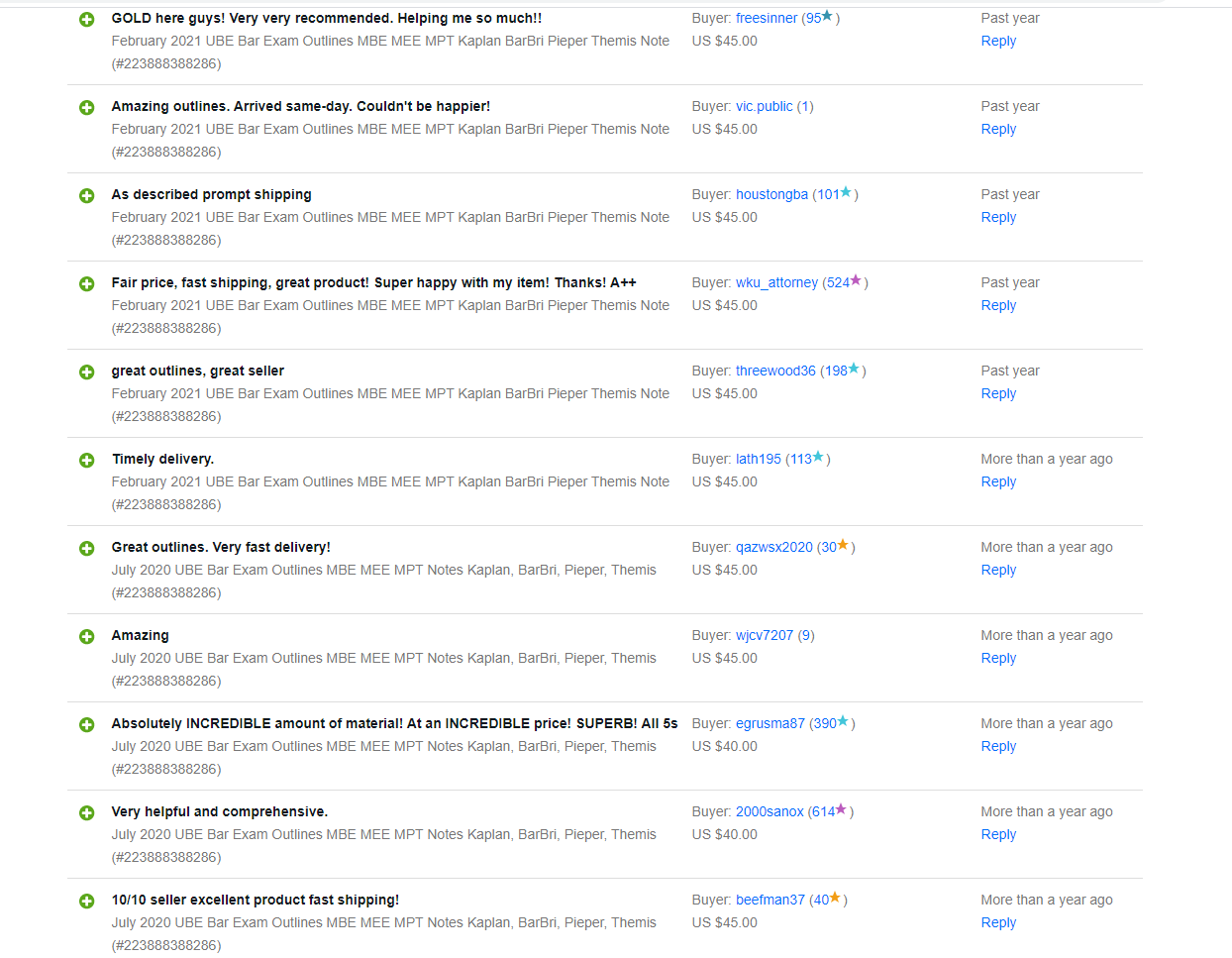A detailed table displays various reviews from buyers in a product store. Set against a white background, the table comprises 11 rows, each marked at the beginning with a green circle containing a white plus symbol. The first column presents the review title in bold black text, followed by the review date and additional information in gray. Dates span from February 2021 to July 2020; rows one through six are February 2021, and rows seven through eleven are July 2020. At the bottom of each row, the review ID appears in gray parentheses, prefixed by a hashtag and a series of approximately 10 digits.

The second column features the review text in gray, the buyer's name in blue, and their star rating in parentheses. For instance, the first row lists the buyer FreeCenter with a rating of 95 and a blue star. While not all buyers have stars, notable entries include the fourth row, which has a rating of 524 with a purple star. Beneath the buyer information, the sale amount is indicated, mostly $45, except for the ninth and tenth reviews, which are $40 each.

The rightmost column details when the review was posted; the first five reviews are labeled "past year" in gray, while the remaining six state "more than a year ago." Below these time stamps, a light blue "reply" link is provided. Thin gray dividing lines separate each row, giving the table a structured layout.